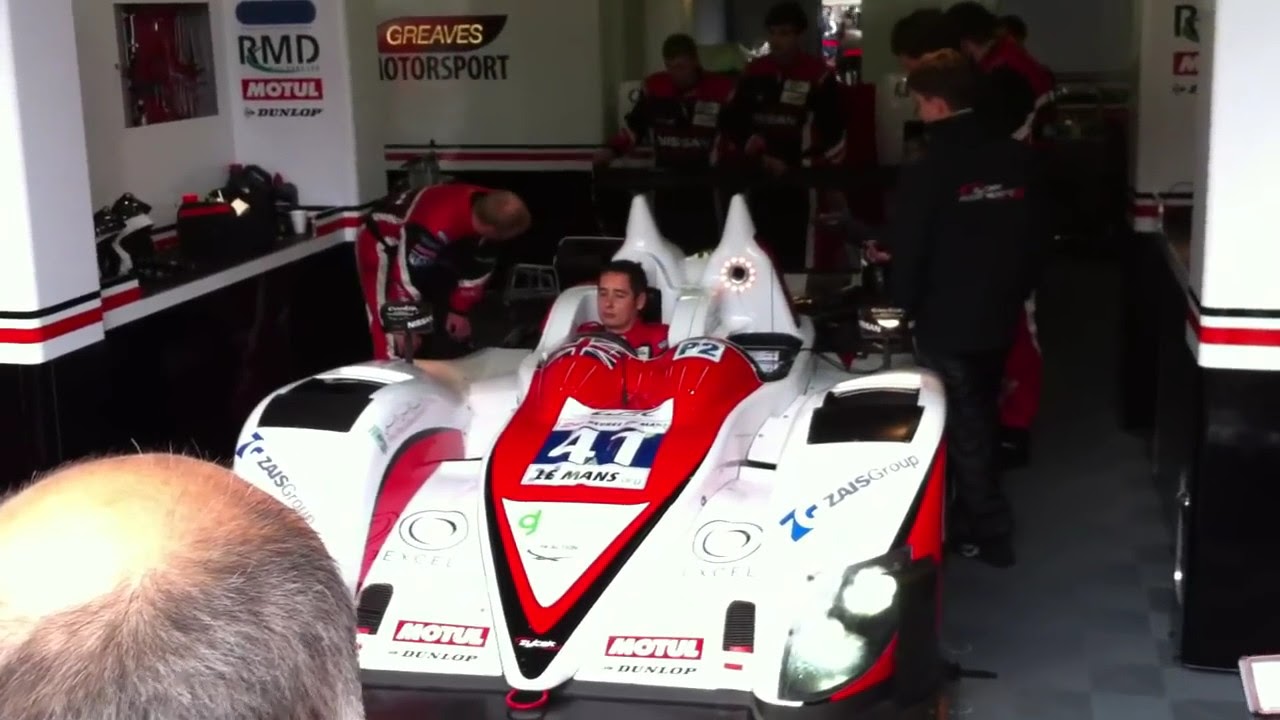The photo showcases a sophisticated, sleek white race car with a distinctive red center, prominently displaying the number 441 and the Le Mans logo. Seated centrally in the driver's cockpit, a man with short brown hair and a red top is visible, although only from the shoulders up due to his low seating position. His expression is neutral, with eyes closed. Around the car, several individuals in red and black racing uniforms cluster, including one bent over the car, while two others appear blurred in the background. The setting reveals a room with black-bottomed, white-topped walls adorned with red and black stripes, featuring writings such as "RMD," "Motul," and "Dunlop," along with the name "Greaves Motorsports." On the left bottom corner, the balding, graying head of another man is partially visible. The room includes columns on the right, a grey tiled floor, and a counter on the left.